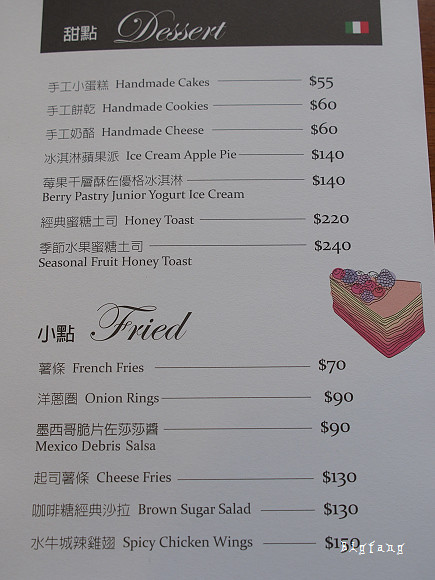At the very top of the image is a black rectangle with cursive white text reading "Dessert" on the bottom left. On the bottom right of this rectangle, there is an Italian flag comprising green, white, and red vertical stripes. 

The menu lists various handmade desserts with their prices, which are likely in another currency that uses the dollar sign. The items and their corresponding prices are as follows:

- Handmade Cakes: $55
- Handmade Cookies: $60
- Handmade Cheese: $60
- Ice Cream: $140
- Apple Pie: $140
- Berry Pastry: $140
- Junior Yogurt: $140
- Honey Toast: $220
- Seasonal Fruit: $240
- Fried French Fries: $70
- Onion Rings: $90
- Mexico Debris Salsa: $90
- Cheese Fries: $130
- Brown Sugar Salad: $30
- Spicy Chicken Wings: $150

On the bottom right corner of the image, there is a watermark with a stylized font that is difficult to decipher. 

In the middle of the image, there is a picture of a slice of cake. The cake features red berries and blueberries on top, a pink section just beneath the berries, followed by alternating yellow and red layers. 

The menu is printed on paper with a shadowed background, giving the entire image a grayish tone. The lighting is not optimal, causing some areas to appear dimly illuminated.